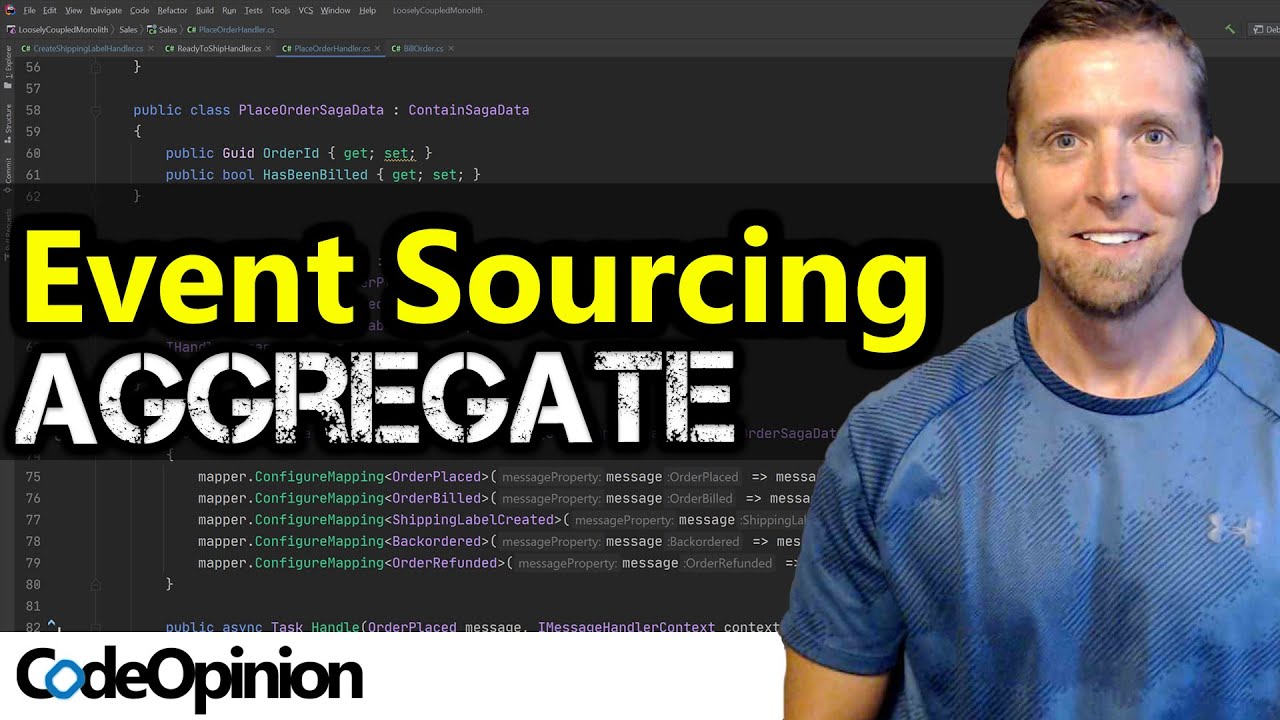A detailed and polished caption for the described image might read:

---

Screenshot of a webpage displaying a section on coding and computer programming. On the right side of the image is a smiling Caucasian man with short hair and a light stubble, dressed in a light blue t-shirt with black designs running over the shoulders. Over his left breast, there is an indistinguishable logo.

The background of the webpage is primarily black, adorned with colorful lines of code in shades of blue, purple, green, white, and gray. Superimposed in the middle of the page is a large caption reading "Event Sourcing" in bold yellow text, with "Aggregate" written underneath in white but weathered text, giving it a worn-off paint effect.

At the bottom of the image, there is a white horizontal band extending to the man’s sleeve, with the branding "CodeOpinion" inscribed in the bottom left corner. The first 'O' in "Code" is a unique, curved diamond shape in blue, while the remaining letters are black. The 'O' in "Opinion" is also capitalized, as is the 'C' in "Code," with the entire phrase written as a single word.

---